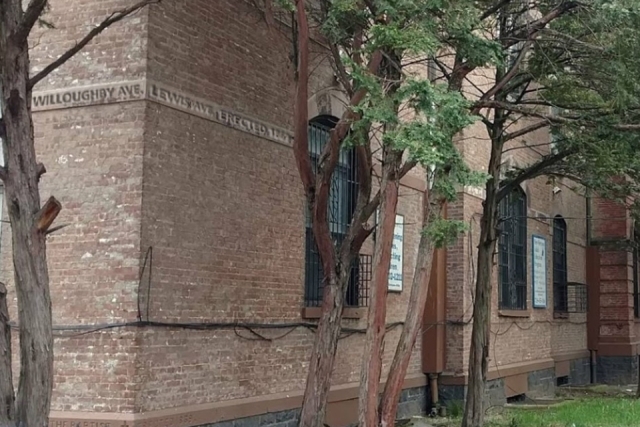This image captures a somewhat gloomy, unremarkable corner of an old red brick building, possibly on a university campus. The building features tall, narrow windows adorned with black metal grates. From the camera angle, you can see both the left and right sides of the structure. The left side, closer in view, showcases a large barred window and is shadowed by a tree with barren branches. Further along the right side, the building extends off the page, displaying additional windows similarly secured with iron bars. 

In front of the building stand four skinny trees with varying amounts of foliage, some bearing green leaves at the top. Nearby, a patch of relatively long grass suggests an untended outdoor area. The bottom quarter of the building is crisscrossed by black cables, and subtle signage appears on the brickwork, though its details are too small to decipher. Above, faint words, "Willoughby Avenue" and "Lewis Avenue," can be made out along the upper molding, along with a partially readable date, lending a slight historical touch to the scene.